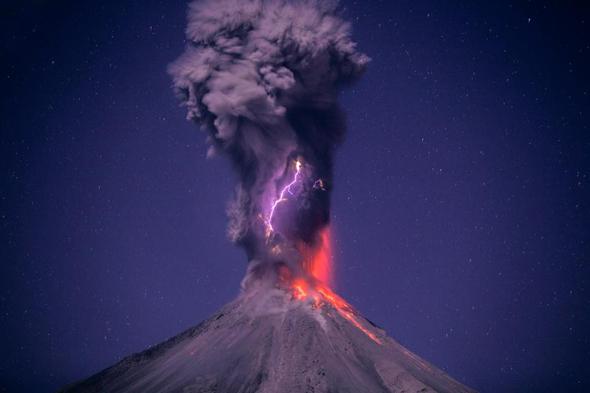The photograph captures a dramatic nighttime eruption of a conical stratovolcano, set against a dark blue and starry sky. The peak of the volcano occupies the center and lower part of the image. The mountain itself is a dark brownish-gray, and it's erupting forcefully, spewing vibrant red lava down its right side. The eruption is explosive, characterized by a massive, billowing plume of smoke and ash that transitions from dark gray at the base to lighter shades higher up. Strikingly, within this turbulent column of smoke, a vivid purple bolt of lightning cuts diagonally upward to the right, adding an electrifying and almost surreal touch to the scene. The sky above is speckled with numerous stars, enhancing the dramatic contrast between the volatile eruption and the serene night.